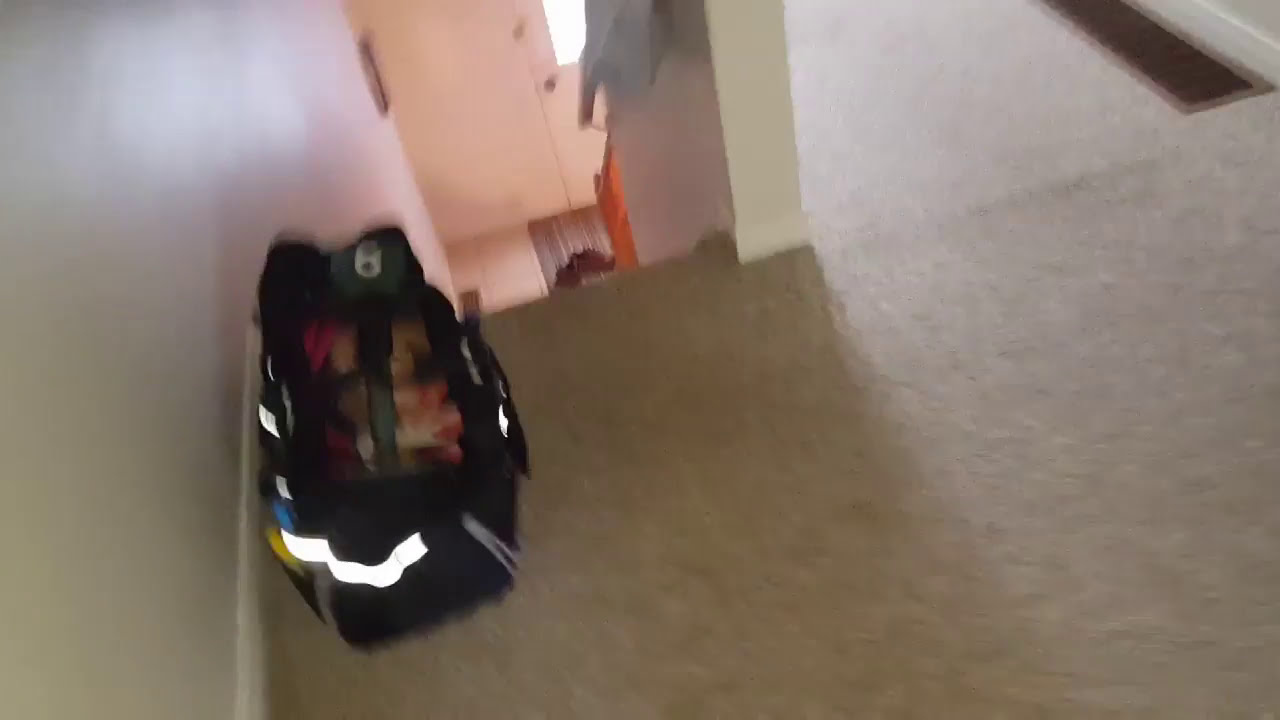At the top of a flight of stairs within a house, there is a landing featuring light green carpet. On the left side of the image, a white wall runs parallel to the landing. At this spot, a black bag adorned with white lines is positioned on the carpet; the bag is open, revealing various colorful items inside. The stairs descend directly from this landing, and at the bottom of the stairway, a window ushers in bright light. On the right side of the landing and extending away from it is a hallway, marked by a floor vent that resembles an air heater opening. The image is slightly blurry, making it difficult to see every detail clearly, but the black bag, possibly a work or sports bag, stands out with its fluorescent white highlights and handle that stretches across the top. The bottom of the stairs appears to have a banister on the right side and leads to what looks like 12x12 porcelain tiles and a rug, indicating proximity to a front door with visible doorknobs.